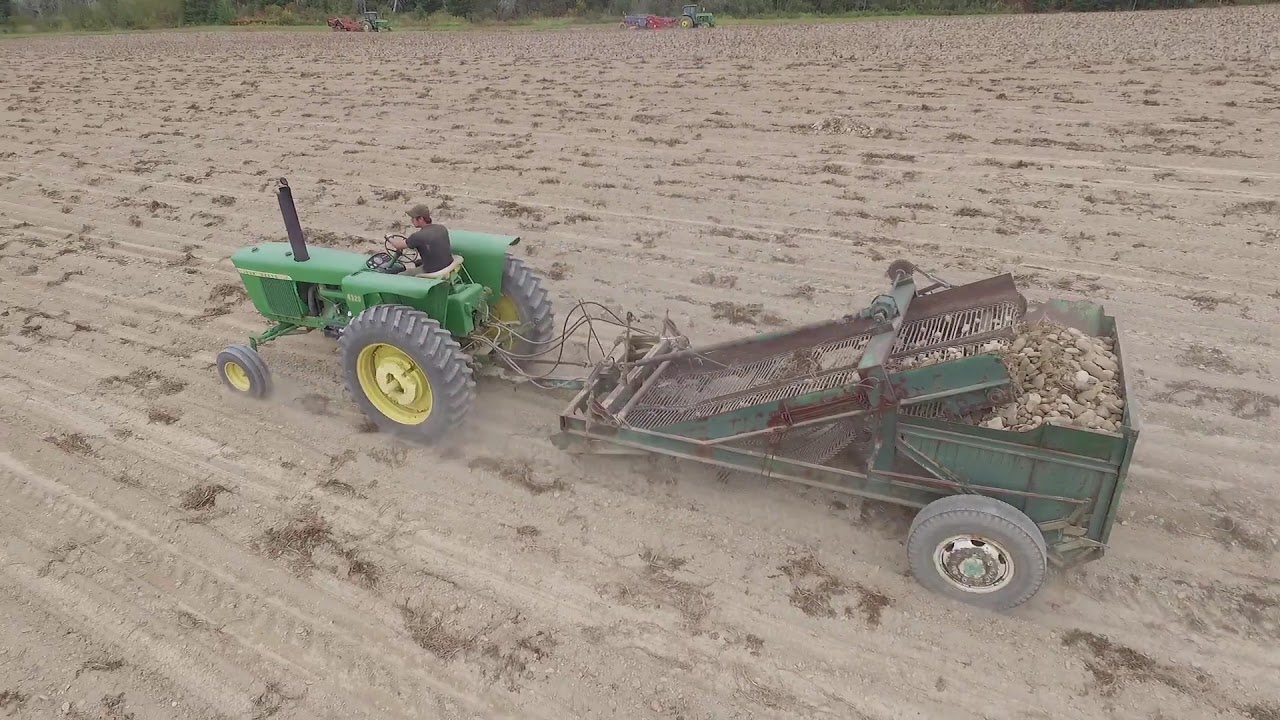The image is a detailed outdoor photograph captured on a clear day. It features a man in a dark shirt and cap, driving a green tractor across a large dirt field situated in the mid-left of the image. The tractor, moving from right to left and slightly upwards in the frame, is towing a piece of farming equipment equipped with a conveyor belt. This equipment appears to be collecting rocks and dirt into an attached wagon, likely in preparation for planting. The foreground reveals evenly spaced tire tracks across the barren soil, indicating systematic field preparation. In the background, near the top of the image, two additional tractors, also green, can be seen heading in the opposite direction. Behind these tractors, a line of trees and green grass marks the edge of the field.